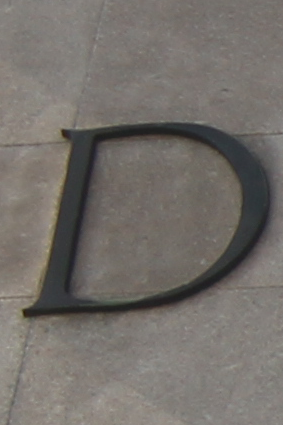The photograph captures a dark gray, stylishly curved, metallic uppercase letter "D" affixed to an outdoor wall. This wall, constructed from pieces of stone in varying shades of gray, brown, and speckled with white and red, is segmented by straight, vertical and horizontal grooves that give a tiled appearance. The letter "D" features a thick vertical stem with a slight jut at its edges, transitioning into the thin, looping curve that widens in the middle before tapering back towards the stem.